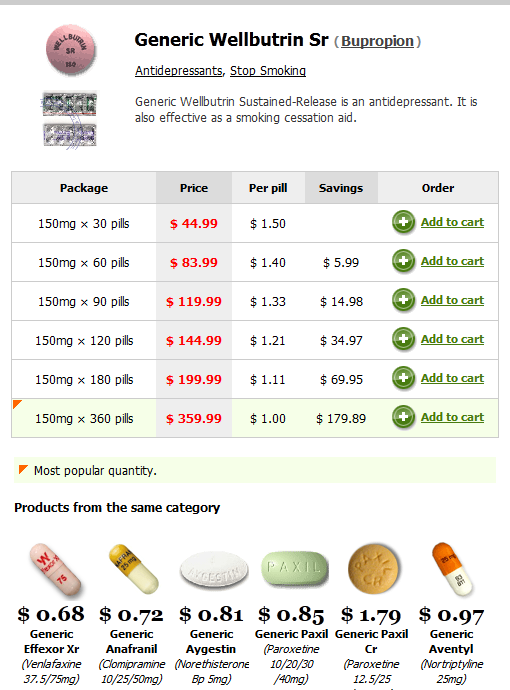The image is a detailed informational page for an antidepressant medication. In the top left corner, there's a close-up of an orange-tan round pill with "Welbutrin" embossed in a circular pattern along the edge, "SR" below the name, and an out-of-focus number underneath. 

To the right of this pill image, the text reads: "Generic Welbutrin SR (Bupropion)", followed by "Antidepressants Stop Smoking". The text clarifies that Generic Welbutrin Sustained Release is not only used as an antidepressant but is also effective as a smoking cessation aid.

Below this, there's a chart with a gray background, featuring five columns labeled: "Package," "Price," "Per Pill," "Savings," and "Order." Under "Package," the chart specifies the dosage and number of pills available, such as 150 mg and 30 pills. The "Price" column lists the total cost in dollars, while "Per Pill" shows the cost per individual pill. The "Savings" column indicates any potential savings in dollars. The "Order" column includes a plus button and an option to add the item to the cart. 

The highlighted option indicates the best value: 150 mg, 360 pills for $359.99, with a price per pill of $1 and savings of $179.89. This option is marked as the "most popular quantity."

Below this chart, there's a section titled "Products from the Same Category," showcasing images of six different pills along with their respective names and prices per pill.